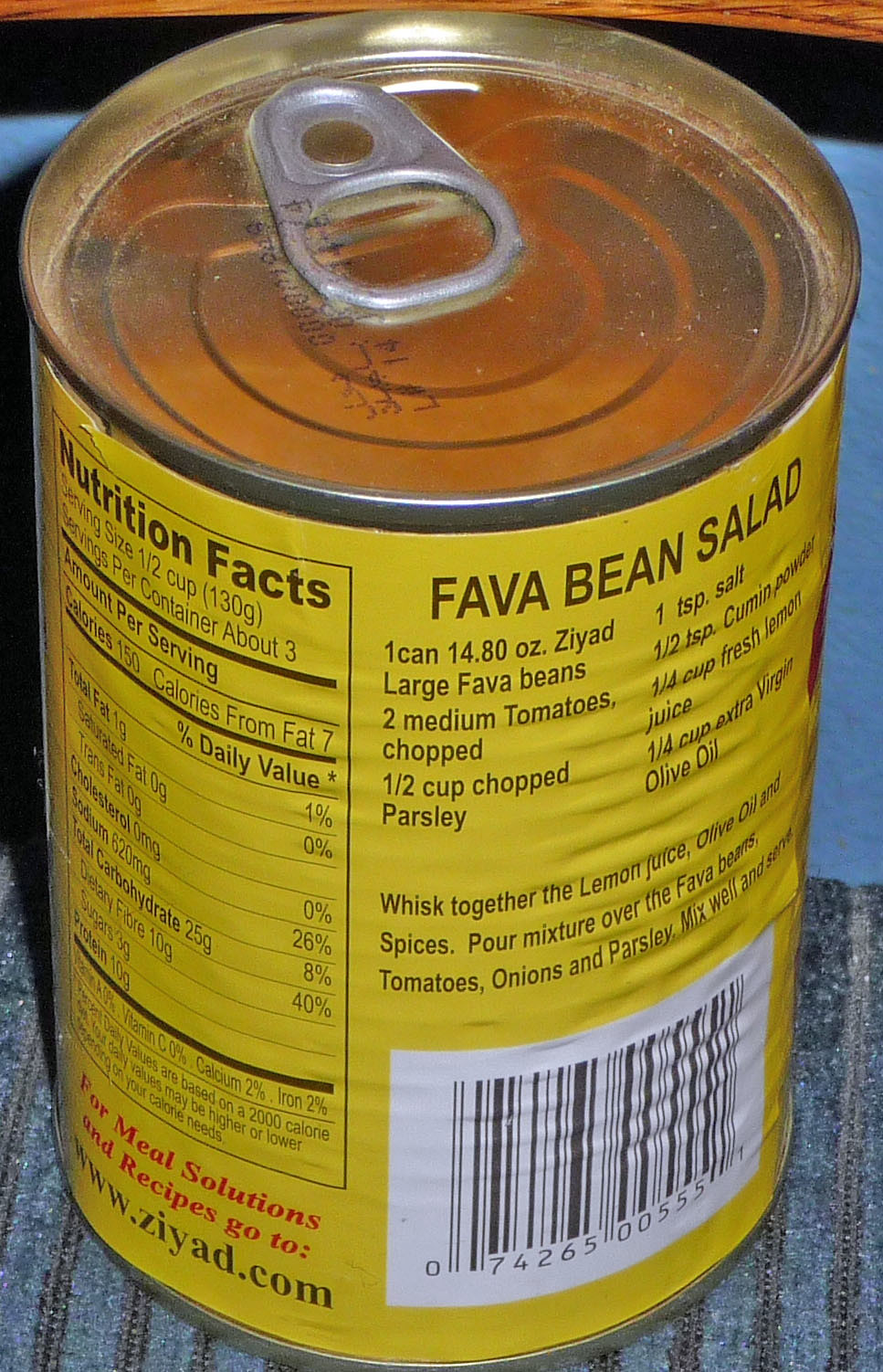This image is a close-up photograph of the back of an unopened, metal can with a pull-tab lid, which appears slightly dirty or old. The can's label, primarily yellow with silver and gold tint, is partially torn at the upper left. The top of the lid has unreadable black stamped letters or numbers.

The yellow background label prominently features the words "fava bean salad" in black lettering on the upper right side, followed by a detailed recipe for the dish: "One can 14.8 oz Ziad large fava beans, two medium tomatoes chopped, half cup chopped parsley, one teaspoon salt, half teaspoon cumin powder, quarter cup fresh lemon juice, quarter cup extra-virgin olive oil. Whisk together the lemon juice, olive oil, and spices. Pour mixture over the fava beans, tomatoes, onions, and parsley. Mix well and serve."

The lower right corner contains a barcode within a white rectangle, and on the bottom left, in red text, it directs viewers to "For meal solutions and recipes, go to www.ziyad.com." Partially visible nutritional facts indicate the serving size as half a cup (130 grams), having seven servings per container. Other nutritional details include 150 calories per serving, with 10 grams of protein, 1 gram of total fat, 0 grams of saturated and trans fat, 620 milligrams of sodium, 25 grams of total carbohydrates, 10 grams of dietary fiber, 3 grams of sugar, and 2% daily value of calcium and iron. Vitamin A and Vitamin C percentages are not legible.

The can rests on a surface with blue and dark stripes, likely a rug or kitchen towel.